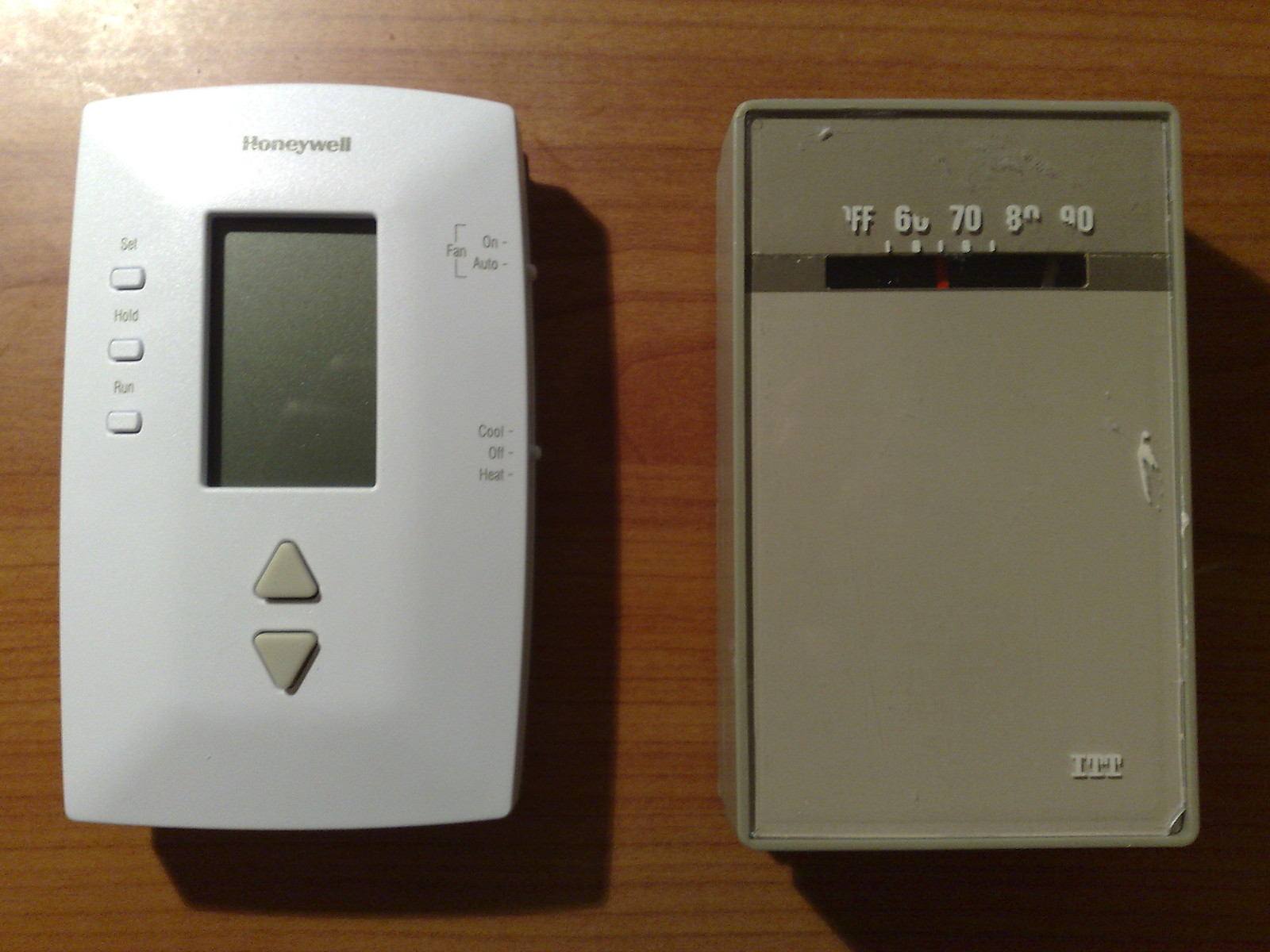This photograph captures a side-by-side comparison of a vintage ITT thermostat and a modern Honeywell thermostat, both mounted on a wood grain surface. The older thermostat on the right exudes a nostalgic charm with its worn exterior and simple design. It features a basic dial with a bar indicator that points to the approximate temperature setting, and a logo in the lower right corner reading "ITT". In contrast, the newer thermostat on the left showcases contemporary functionality and sleek aesthetics. With a light gray or off-white finish, it includes an LCD display and various buttons labeled "fan control on or auto", "cool, off, heat", "up", "down", "set", "hold", and "run". The brand name "Honeywell" is prominently displayed above the display. The juxtaposition of these thermostats illustrates the evolution of home heating technology, highlighting the advancements in user interface and control precision.